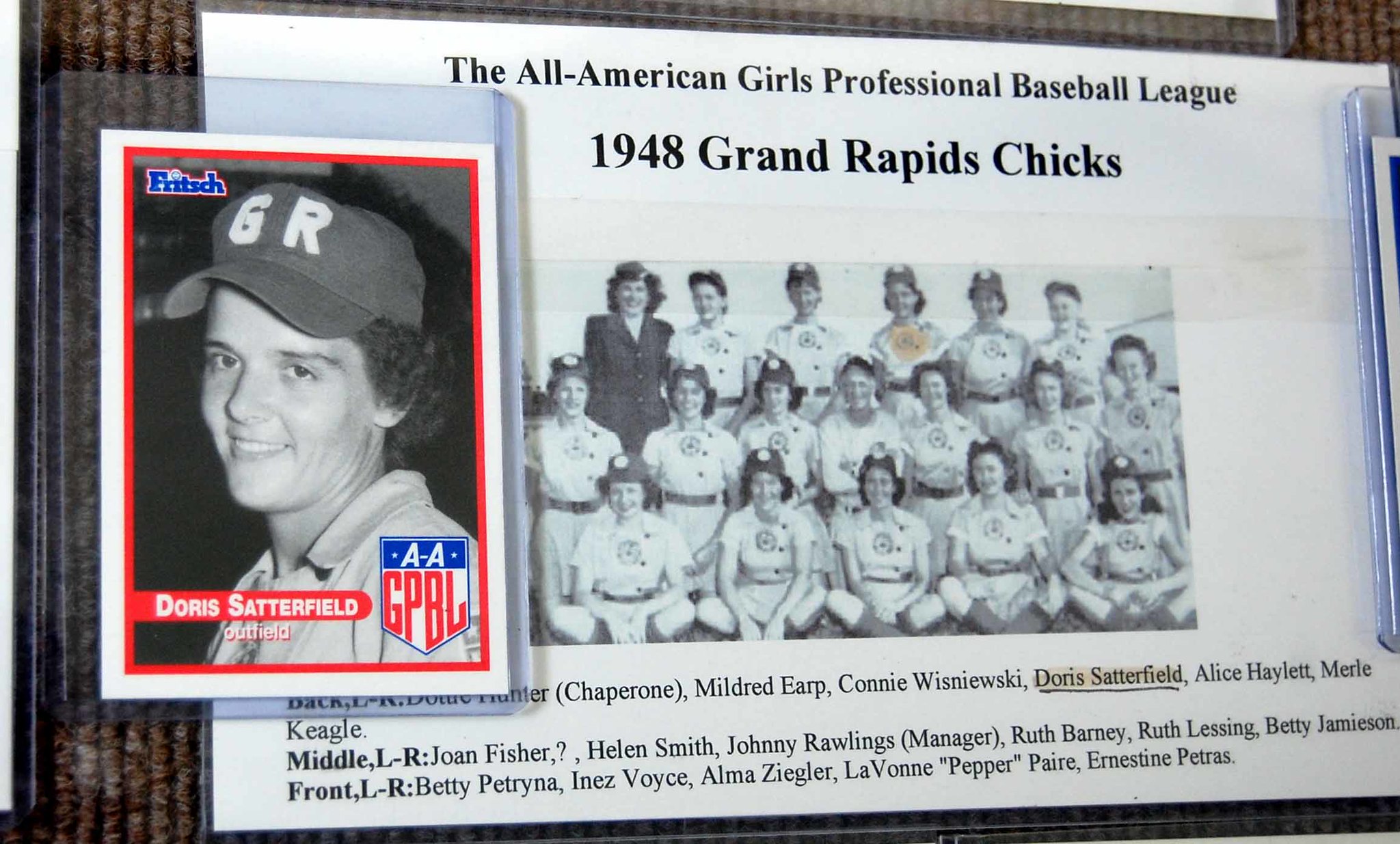The image is a detailed photograph showcasing memorabilia from the All-American Girls Professional Baseball League (AAGPBL). On the left side, a vintage baseball card features Doris Satterfield, an outfielder for the 1948 Grand Rapids Chicks. The card, encased in plastic, displays her name and position, with a distinct red and white border and "GR" for Grand Rapids on her hat.

To the right of the card lies a white piece of paper. At the top, bold black text reads "The All-American Girls Professional Baseball League, 1948, Grand Rapids Chicks." Below this heading is a black and white team photograph, neatly arranged in three rows: the first row of players sits cross-legged, the second row kneels, and the last row stands. In the upper left corner of the team photo, the coach is visible.

Doris Satterfield's name is notably underlined and highlighted in the team roster beneath the picture. The names of all the players are listed, detailing their positions from back to front row, left to right. The photograph is set against a brown, twilled rug, emphasizing the historical and cherished nature of the memorabilia.